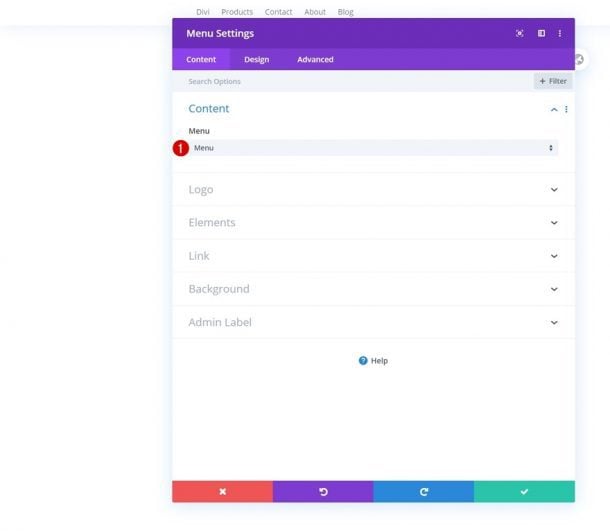The displayed web page is a settings menu for a program. At the very top, there is a navigation bar with options including "DvProducts," "Contact," "About," and "Blog" presented in gray text. Beneath this is a prominent purple bar, with the "Contacts" menu located on the far right and an option to expand.

The main settings menu is displayed with white lettering on a purple background and includes three primary tabs: "Content," "Design," and "Advanced." Directly below these tabs, there are search options and a filter button situated to the far right. 

The "Content" tab is highlighted in blue and features a pull-up context menu. Within this menu, there is an item labeled "Menu," again presented in a context menu format. Accompanying this is a red circle containing the number "1," indicating a notification or alert.

Additional menu items listed include "Logo," "Elements," "Link," "Background," and "Admin Label," each of which has its own context menu.

At the bottom of the menu are four colored blocks: a red block with a white "X," a purple block with a refresh icon, a blue block with another refresh-style icon, and a green block with a white check mark. These buttons likely serve various functions such as closing, refreshing, or confirming actions within the menu system.